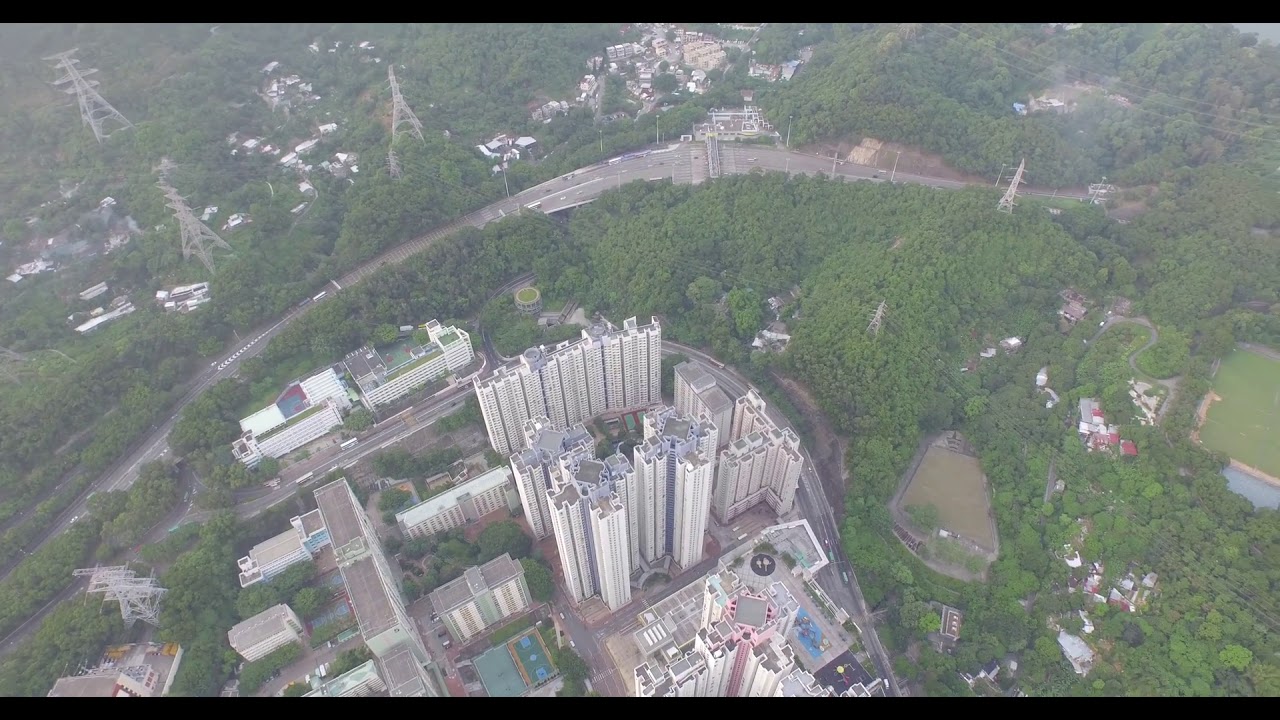The aerial image provides a stunning bird's-eye view of a cityscape partially surrounded by dense greenery. From what appears to be the vantage point of a drone or helicopter, about 50%-60% of the landscape is dominated by lush trees, creating a stark contrast with the urban area. In the lower half of the image, from the middle towards the bottom left, lies a semi-circular cluster of high-rise residential buildings. There are approximately 18 to 20 tall, white structures, each around 20 to 30 stories high, some arranged in rows while others are interspersed amongst smaller buildings. These high-rises share a uniform design, notably shaped like a plus sign, suggesting a cohesive architectural plan. The urban area is bustling but appears to be well-integrated with nature, featuring several electrical wire towers and small pockets of neighborhood activity visible amidst the vegetated surroundings. This harmonious blend of urban and natural elements encapsulates a vibrant community with a serene, green environment.